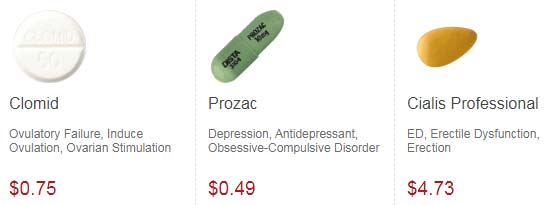This image is a cropped screenshot from a pharmaceutical website showcasing three medications. Each medication is presented in a square box format. At the top of each box, there's a photo of the medicine's front view. Below the images, the names of the medications are displayed in large gray fonts. Further down, each description outlines the conditions the respective medication treats. Finally, at the bottom left of each box, the price per pill is stated in large red font.

The first medication features a large white pill labeled "Clomid." Its description states that it is used for ovulatory failure and induction ovulation of ovarian stimulation. The price per pill is noted as $0.75.

In the center, an angled photo of a green capsule labeled "Prozac" is shown. This medication is identified for treating depression, serving as an antidepressant, and addressing obsessive-compulsive disorder (OCD). The price per pill for Prozac is $0.49.

The last medication on the right is a yellow pill shaped like a sunflower seed, labeled "Cialis Professional." Its description specifies that it is used for erectile dysfunction (ED) and erection-related issues. The cost per pill for Cialis Professional is $4.73.